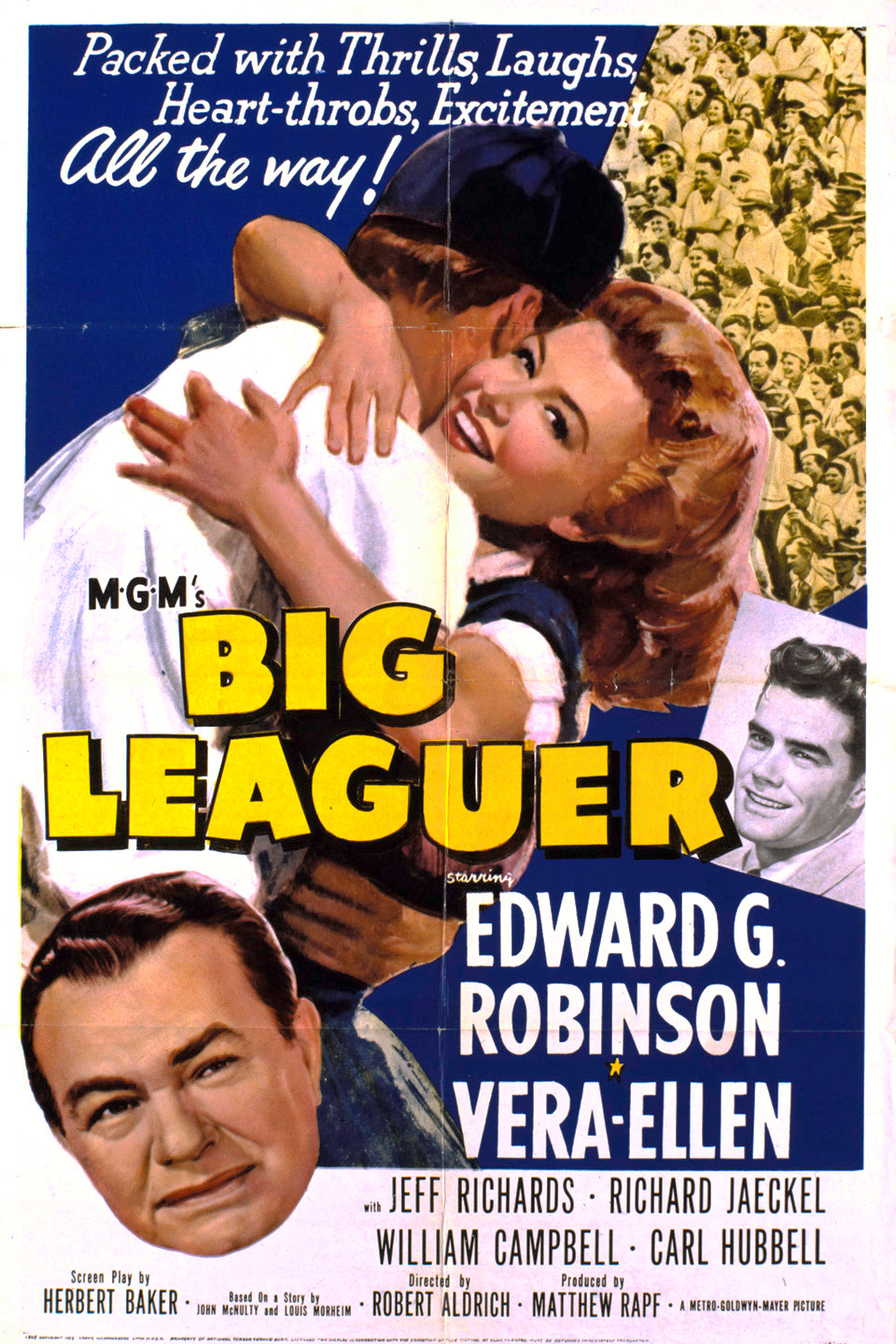The poster exhibits a vibrant 1940s or 1950s style, featuring a central visual of a joyful, Caucasian blonde woman with reddish-brown hair smiling at the camera as she embraces an unseen man wearing a blue cap and white shirt, hinting at an athletic, possibly baseball-themed storyline. Behind her, a detailed crowd adds depth without focusing on any one individual. The top left corner contrasts with a navy blue background and white text that reads, "Packed with thrills, laughs, heartthrobs, excitement all the way!" Dominating the composition is bold, yellow text proclaiming "MGM's Big Leaguer," with white text beneath naming the stars, Edward G. Robinson and Vera Ellen. Supplementary pictures in the lower part feature two men: one mid-40s with black hair, and another slightly older, in his 50s, with brown hair. Additional names mentioned include Jeff Richards, Richard Jekyll, William Campbell, and Carl Hubbell.